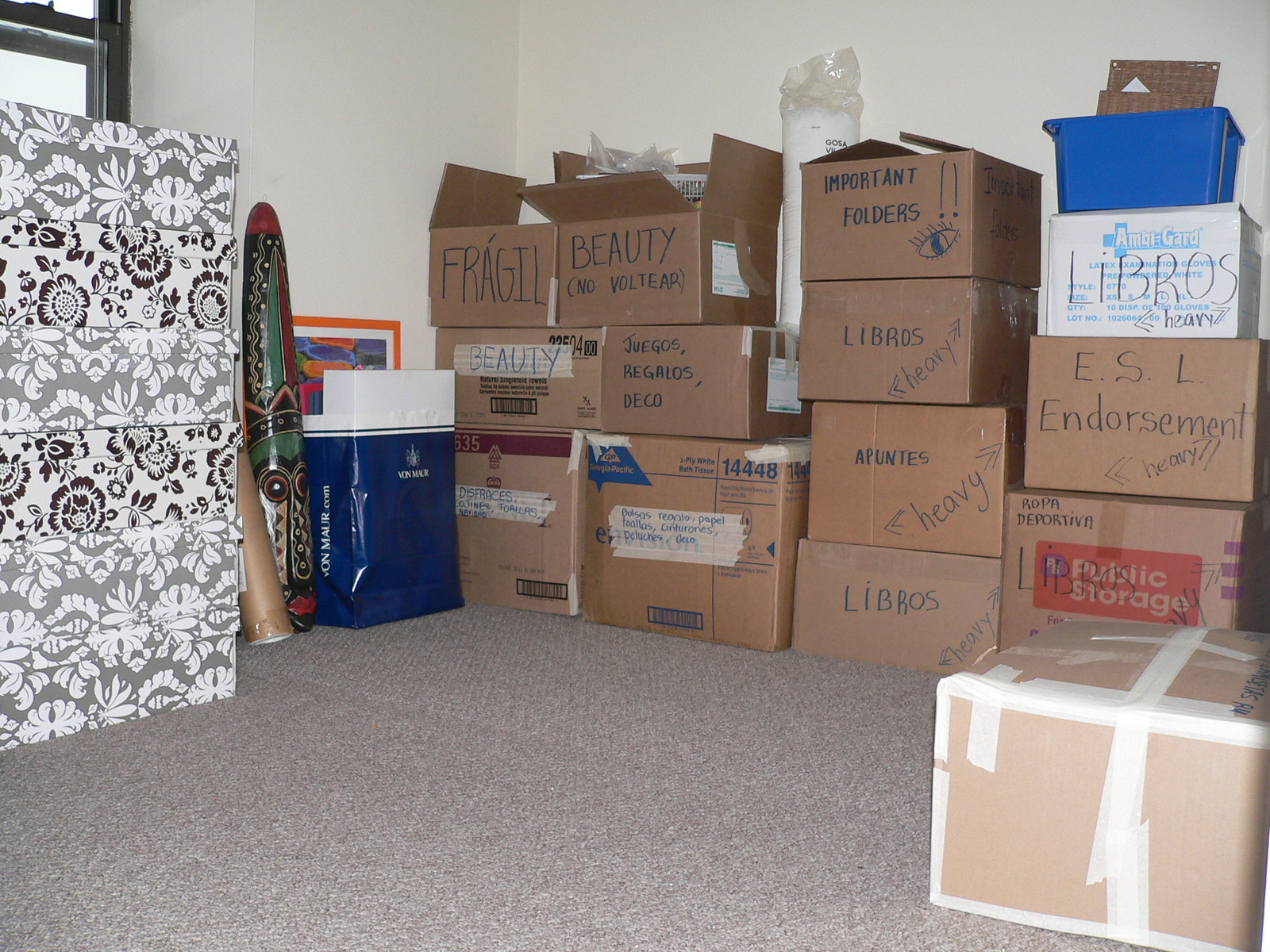The photograph captures a cluttered room, possibly within a house or commercial building, characterized by its gray carpet and white walls. In the upper left-hand corner, a black window is partially visible. The room is filled with an assortment of brown cardboard boxes, some tagged with blue text bearing descriptions such as "Important Folders," "Libros (Heavy)," "ESL Endorsement (Heavy)," "Fragile," "Beauty," "Juegos, Regalos, Deco," and others that lack labels or feature decorative patterns. Notable among the items is a large blue and white bag on the left side marked "VAMAR, Van Muir," situated next to what appears to be an artifact of Indian or Asian origin. Adjacent to this artifact is a brown cardboard tube and a stack of boxes with black and white or gray and white floral designs. Some of the boxes are partially open, adding to the disordered appearance of the space.